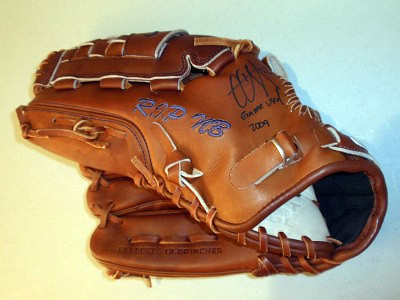This photograph captures a close-up of a medium brown leather, right-handed fielder's baseball glove, positioned on its side from left to right. The glove, featuring rawhide lacings and white stitching, is displayed against an unusual background with a gradient that transitions from light yellow to light blue, possibly due to unique lighting conditions. On the glove, the stitched words "RAPMB" are prominently visible, accompanied by a signature in black ink. Beneath the signature, the phrase "Game Used 2009" is clearly inscribed, adding a touch of historical significance to the image.